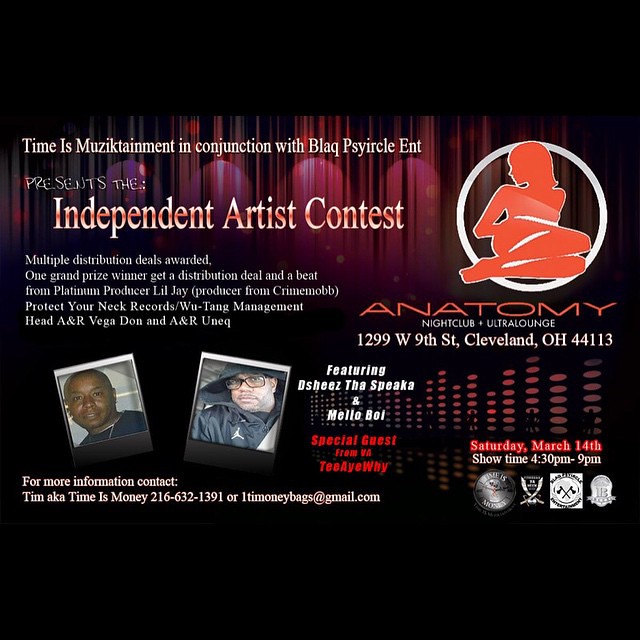On a predominantly black background, this concert promotion poster prominently features white text with some splashes of red. At the top, in white print, it reads, "Time is Music Entertainment in conjunction with Black Cycle Entertainment", heralding an "Independent Artist Contest". Below this text is a red and white silhouette of a woman leaning down with her legs folded, framed by a circle.

The poster promises attractive benefits for participants, stating, "Multiple distribution deals awarded. One grand prize winner gets a distribution deal and a beat from platinum producer Lil’ James, producer from Crime Mob. Protect Ya Neck Records, Wu-Tang Management, head A&R Vegadon and A&R Unique.”

Two photos of artists are slanted just below the central text; on the left is a black artist, and to his right, another artist wearing a brown jacket. The event is labeled with further details, including: "Anatomy Nightclub Ultra Lounge, 1299 West 9th Street, Cleveland, Ohio," and is scheduled for "Saturday, March 14th, showtime 4:30 to 9 p.m."

Highlighted appearances include "Featuring: Deej the Spica and Mellow Boy, with special guest Treatway.” The poster also includes various sponsor symbols at the bottom and provides contact details for further information, listing "Tim, aka Timeismoney" with a phone number and email.

The entire advertisement is framed by dark, almost imperceptible red curtains, accentuating the dark, atmospheric theme of the event.